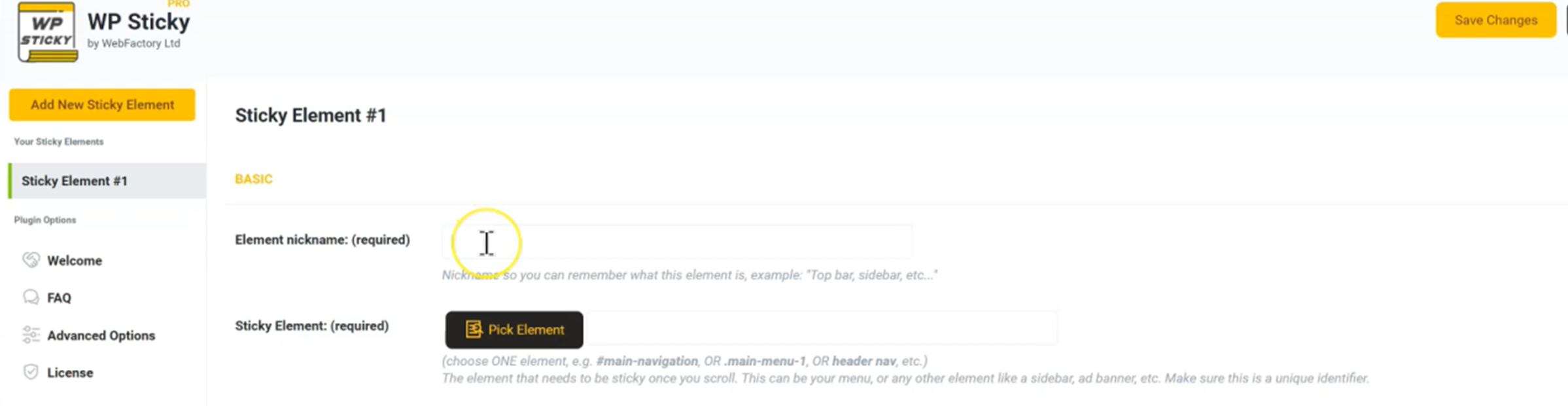The image showcases the interface of the WP Sticky website. In the top left corner, the logo "WP Sticky" is prominently displayed. The interface features a vertical menu on the left side with several clickable tabs: "Add New Sticky Element," "Sticky Element Number One," "Welcome," "FAQ," "Advanced Options," and "License."

To the right, the interface highlights a section labeled with the number "1" and titled "Basic." Underneath, it prompts the user to enter the "Element's Nickname" in a required field, which is currently empty. Following that, another required field labeled "Sticky Element" is displayed. Below this, there is a prominent black button with the text "Pick Element" in bright orange letters. A light gray paragraph of instructional text is present beneath the button, although the text is not legible.